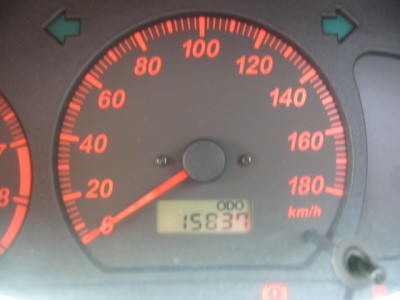The image showcases a speedometer against a blurry, dark gray background. The speedometer's outline is black, with orange graduations and numbers, and an orange indicator hand currently pointing at zero. The gauge ranges from 0 to 180 kilometers per hour. In the center of the speedometer, there is a rectangular counter displaying the numbers "15837," likely representing the total kilometers traveled. At the top of the image, there are two arrows: a pale green arrow on the right, pointing right, and a darker green arrow on the left, pointing left. On the extreme left edge of the image, part of another dial is visible, although its function and details are not clear.